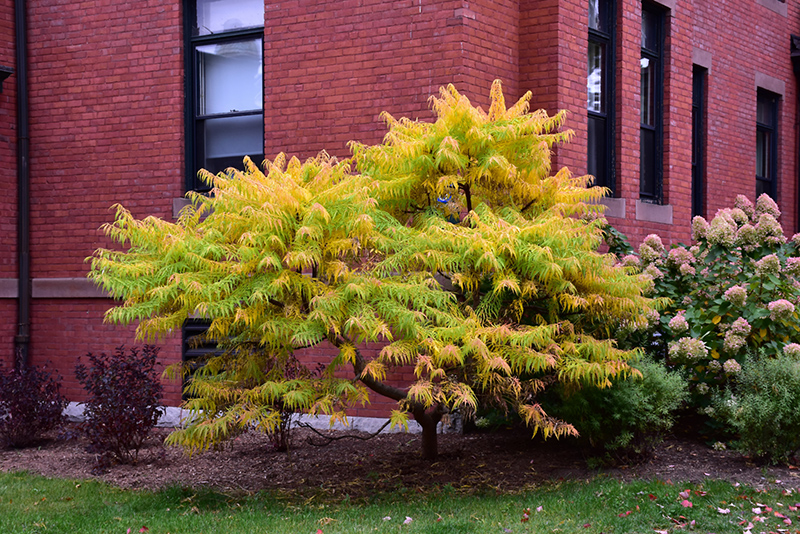This detailed photograph captures a deep red brick building that serves as the backdrop, displaying multiple large windows with black frames and one window featuring a white curtain. The building has a unique design with an indentation on the right side where the windows extend out, and includes a whitish tan border across the bottom along with a black drainage pipe. The scene is set during the fall, evidenced by vibrant leaves scattered on the green grass.

In the foreground, there is a vivid array of foliage. Centrally, a tree with leaves in various stages of color change—some bright green, others pink, and yellow—stands out, adding a dynamic burst of autumn hues to the scene. To the left, two small bushes exhibit a reddish tint, while on both sides of the central tree are two more substantial bushes or trees with thick stems and yellowish-green leaves. Amongst the plants, hibiscus and hydrangeas are clearly visible, contributing to the colorful display with the hydrangeas showing a mix of lime green and pink. The entire arrangement is set within a mulched area, interspersed with wood chips and grass, enhancing the whimsical, seasonal vibe of the photograph.